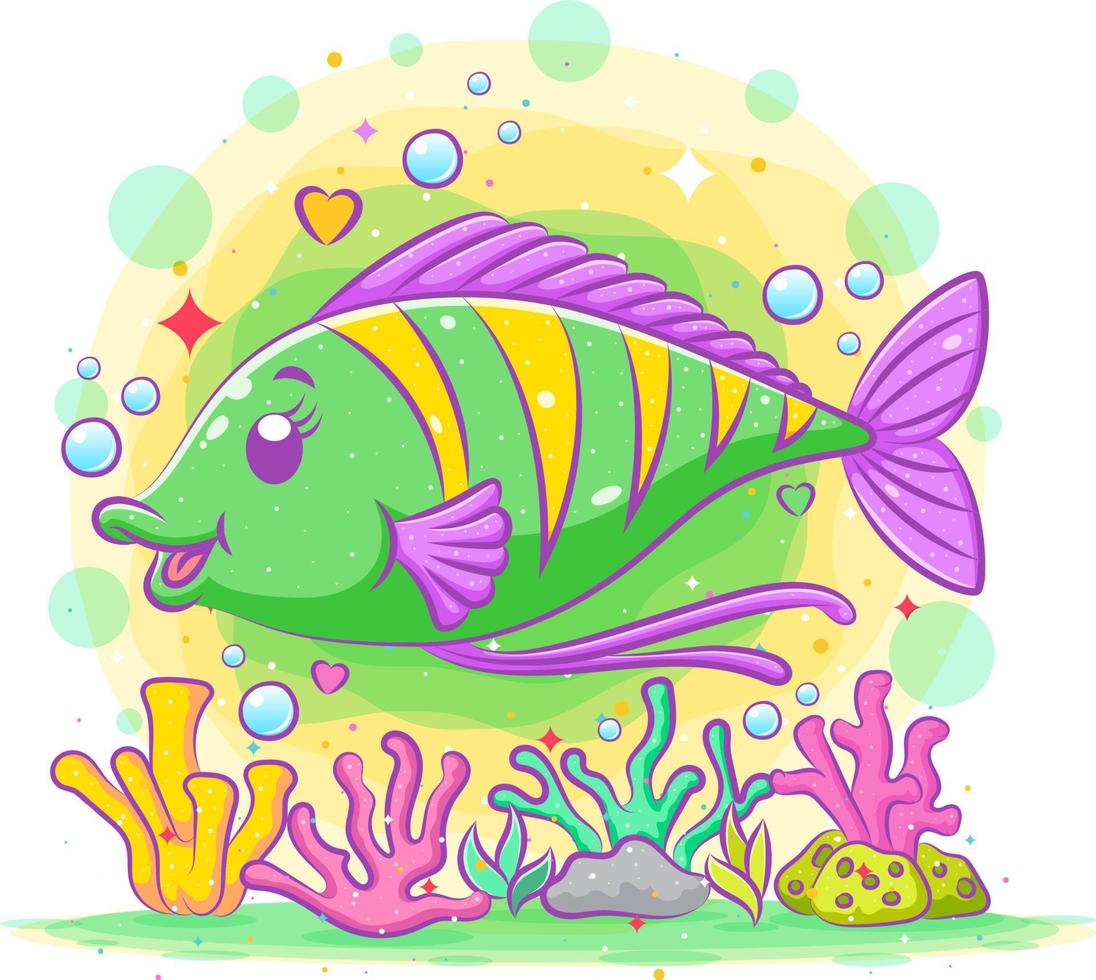This image is a vibrant piece of artwork depicting a cartoon fish set against a white background, typical of a coloring book style. The fish, painted in a lively green, features distinctive accents: purple eyes, lips, and fins, with yellow scales outlined in purple. The inside of its open mouth reveals a pink hue and a hint of a red tongue. Complementing the fish are yellow and green swirls behind it, along with various colored bubbles—blue, green, and yellow. Notably, there is a yellow heart outlined in purple and a red diamond among the bubbles. Beneath the fish, representing the ocean floor or an aquarium setting, is an array of colorful coral: yellow, pink, and turquoise, each accompanied by sections of green plant life and rocks. The scene feels dynamic and cheerful, with the fish and the underwater elements appearing in a vibrant, floating assemblage.